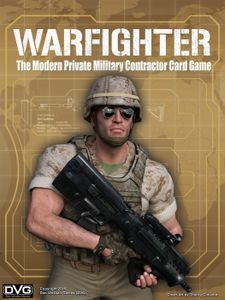This is an advertisement for the card game "Warfighter: The Modern Private Military Contractor Card Game" by DBG. The central image features a muscular soldier wearing a brown and beige camouflaged helmet, reflective aviator sunglasses, a tactical vest in dark green and brown, a short-sleeve rolled-up t-shirt, beige pants, and fingerless gloves. He is holding a large black gun. In the background, there's a faint computer diagram overlay on a taupe and olive green backdrop. At the top of the image, the title "Warfighter" is prominently displayed in all caps, while the bottom left corner includes the brand name "DVG." The image also contains small, unreadable text at the bottom, likely copyright information. This visually striking cover emphasizes the intense, modern military theme of the card game.